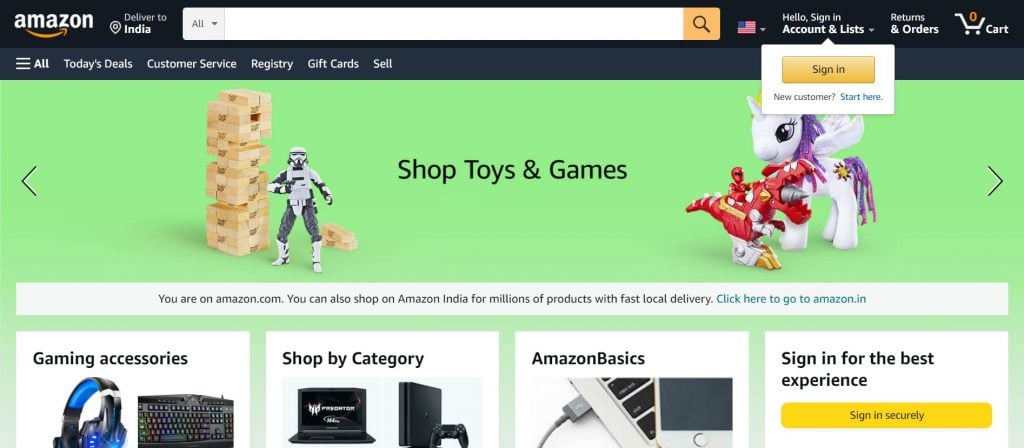This is a detailed screenshot of the Amazon homepage, highlighting various elements:

In the upper left corner, the Amazon logo is displayed in white text, accompanied by the iconic yellow half-smile arrow logo. Below it, the phrase "Deliver to India" is written in white text. Adjacent to this section on the right is the search bar. The search bar features a drop-down menu labeled "All" in black text, followed by a white text box where users can type their search queries. To the right of the text box is a yellow search button featuring a black magnifying glass icon.

Next to the search bar is an American flag icon. Following the flag icon, the text "Hello, Sign in Account & Lists" is displayed in white, with a drop-down menu activated below it. The drop-down menu reveals a white box with a gold bar labeled "Sign in" in black text. Beneath the gold bar, there is a text prompting new customers with "New customer? Start here" in white text.

Further along, the banner features the text "Returns & Orders" in white, and to its right, a white shopping cart icon with a yellow zero inside.

Beneath the main navigation bar, there is a promotional gray box. This box features a Jenga tower, a Transformer robot, and text in black stating "Shop Toys and Games." To the right, there's a red and gray dinosaur figure, a red figure riding it, and a gray unicorn pony with wings and purple hair and tail.

Adjacent to this section, a white box states, "You're on Amazon.com. You can shop on Amazon India for millions of products with fast local delivery" in black text. Below this message, the text "Click here to go to amazon.in" is written in blue.

Towards the bottom, four white boxes provide additional navigation links. These links read: "Gaming Accessories," "Shop by Category," "Amazon Basics," and "Sign in for the best experience" in black text. Below these links, a gray and yellow bar offers another sign-in option with the text "Sign in" in black.

Overall, the screenshot primarily highlights navigation and promotional elements designed to facilitate user engagement and seamless shopping.